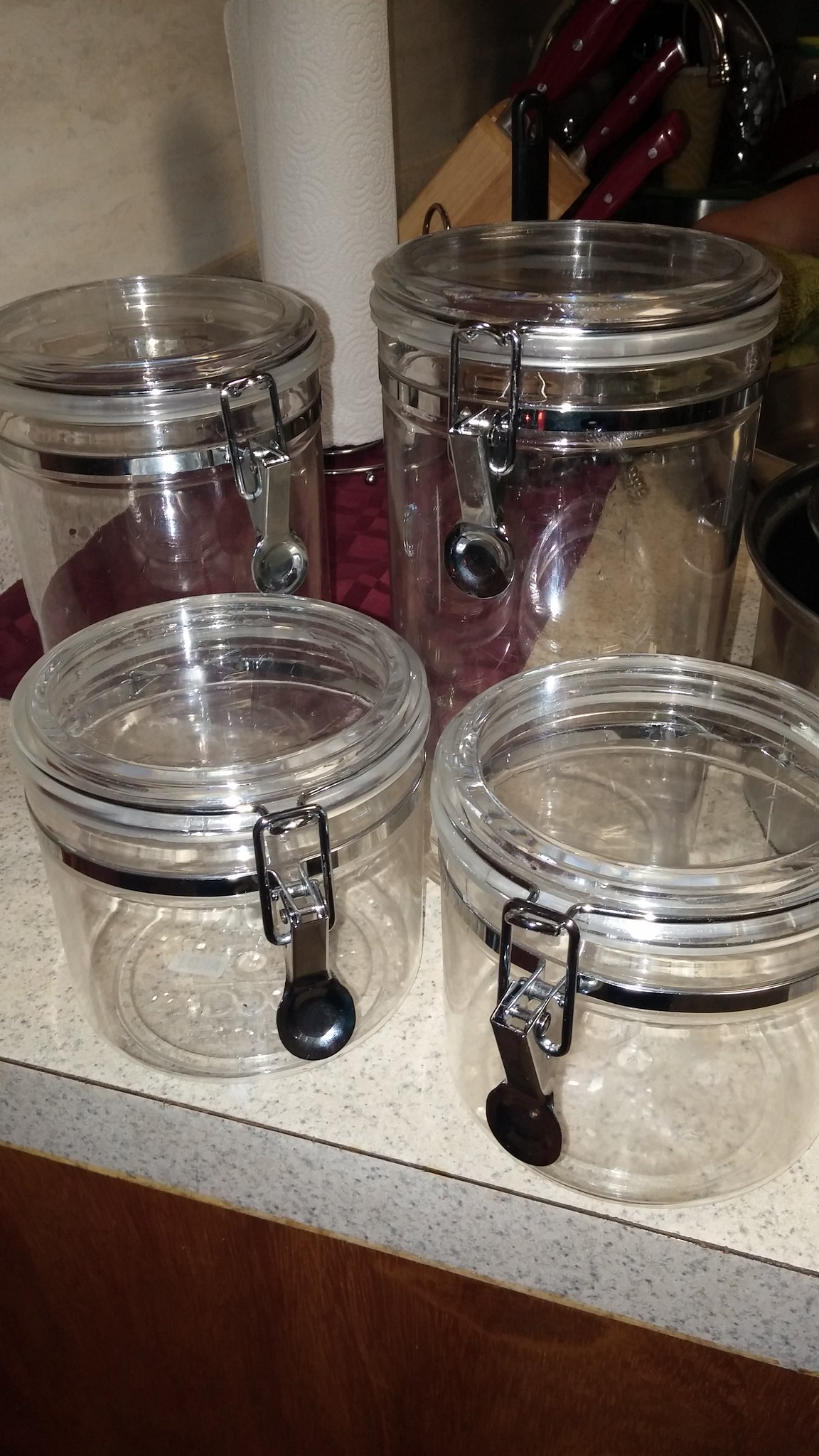In this color portrait photograph taken indoors, we see four glass cookie jars of varying sizes arranged on a white marble countertop speckled with black and gray. Two identical short and squat jars are positioned at the front, and behind them stand two taller jars of similar design. Each jar features glass lids with metal clasps equipped with measuring spoons that hang down from circular serving spoon bases, ensuring a tight seal. The countertop also includes a maroon-colored tablecloth partially extending across it. To the right, there is a light brown knife block housing maroon-handled knives secured with silver metal rivets, along with a silver metal paper towel holder with a roll of paper towels. A black handle, likely part of a kitchen appliance, is visible behind the largest cookie jar, and the upper right corner of the image might show faint details of kitchen sink fixtures amidst the subdued lighting.